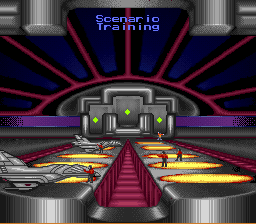This image is a detailed screenshot from a retro-style, low-resolution video game, likely from the MS-DOS era. The scene is set in a futuristic military spaceport or hangar designed for fighter jets or spaceships, featuring a highly metallic environment with elaborate decorations. At the top of the screen, blue text reads "Scenario Training." The background is a large dome, adorned with crimson and red rays radiating outwards, which gives a unique, almost celestial aesthetic.

Scattered throughout the hangar, various spaceships or space fighters are parked on yellow circular landing pads that emit a soft light. Pilots, identified by their black pants and red shirts, are positioned near the spacecraft and along the runways, with some signaling or standing by the sides. The color palette of the scene includes dominant hues of gray, pink, and purple, enhancing the futuristic and metallic feel of the environment. Overall, the intricate design and numerous details create an immersive, visually rich setting.